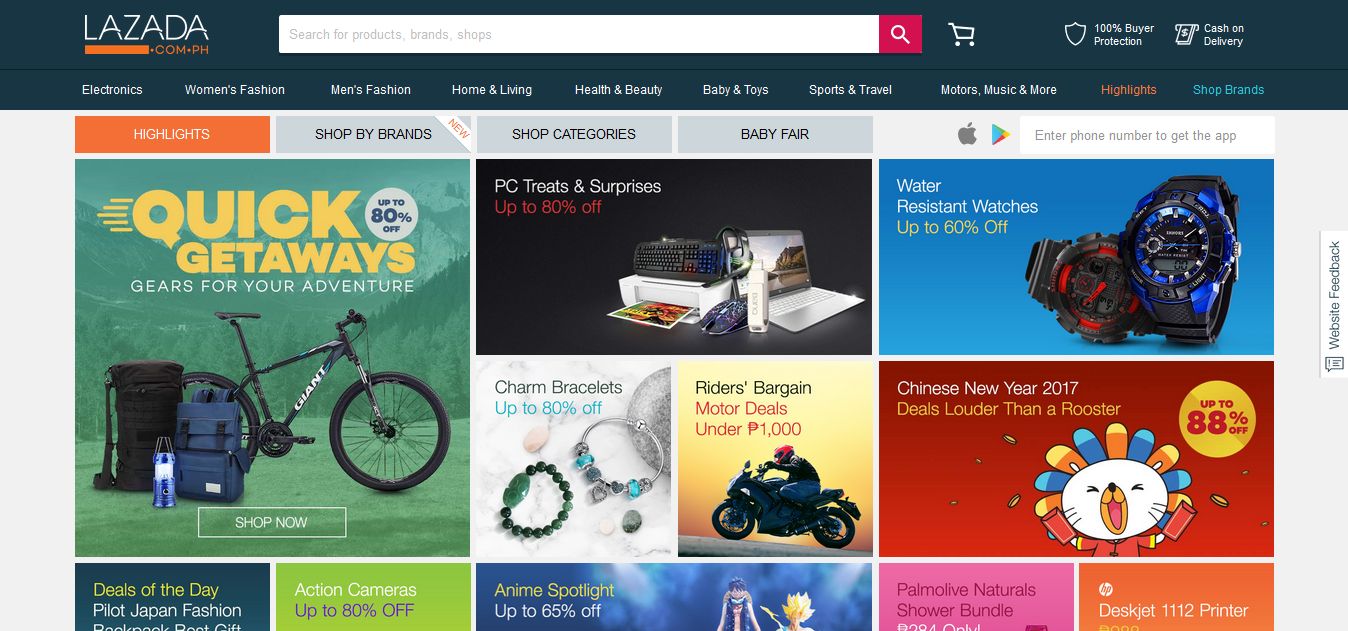The image displays a webpage designed in a style reminiscent of Amazon's interface, featuring a familiar layout and structure. The top of the webpage showcases a navy blue header with the logo "lazada.com.ph" situated in the upper left corner. Adjacent to the logo, there is a prominent search bar accompanied by a shopping cart icon. Key features such as "Buyer Protection" and "Cash on Delivery" are highlighted in the upper right corner.

Directly below the header, a series of category links are displayed, including "Electronics," "Women's Fashion," "Men's Fashion," "Home and Living," "Health and Beauty," "Baby and Toys," "Sports and Travel," "Motors," "Music and More," and "Shop Brands." The "Highlights" section is currently active, offering various promotional items and deals.

Highlighted promotions include:
- **Quick Getaways**: Features gear for outdoor adventures, including a mountain bike.
- **PC Treats and Surprises**: Offering up to 80% off on laptops and computer gaming items.
- **Water-Resistant Watches**: Discounts up to 60% on various watch models.
- **Chinese New Year 2017**: Deals under the theme "Louder than a Rooster."
- **Charm Bracelets**: Reduced prices up to 88%.
- **Writer's Bargains**: Special offers related to writing.
- **Motor Deals**: Vehicles and related accessories priced under $1,000.

The webpage is a detailed and vibrant marketplace bearing a strong resemblance to the Amazon platform, both in its visual styling and functional layout.